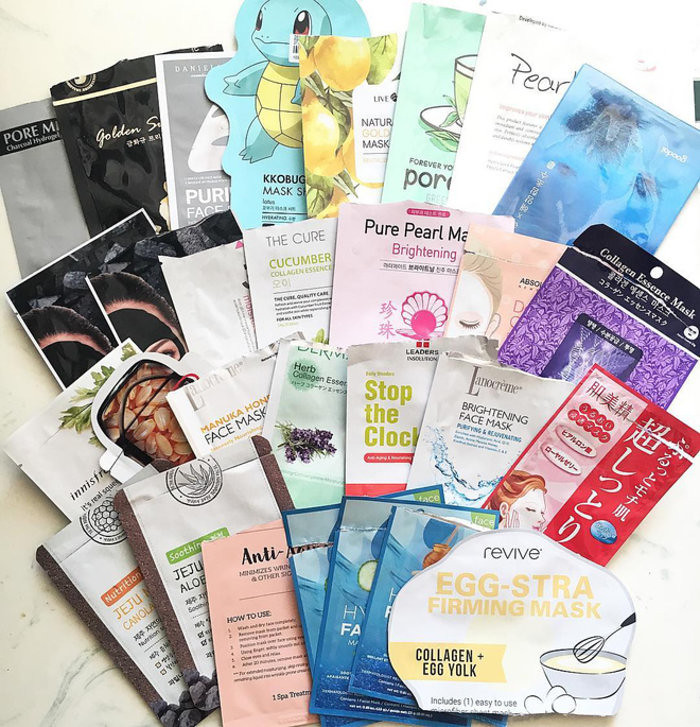The image showcases a diverse collection of self-care products, meticulously arranged on a sleek white marble counter, subtly veined with intricate grey streaks. The focal point is an assortment of around 30 different facial masks, each distinct in design and purpose. Prominently displayed in the front is a mask labeled "Revive," advertised as an "Egg Stra Firming Mask," enriched with collagen and egg yolk, complete with an illustration of eggs being whisked in a bowl. Peeking from underneath are a few blue-packaged masks, their labels obscured, yet their presence adding to the eclectic mix.

Among the standout products, there's "Zhu Zhu," available in both green and orange packets, promising unique benefits. Another captivating mask, "Stop the Clock," implies an anti-aging formula. One has enigmatic Chinese characters, hinting at traditional ingredients or techniques. For those seeking luminosity, a "Brightening Face Mask" serves as an enticing option. Adding a playful touch, a mask with an anime-style turtle graces the spread, alongside a "Collagen Essence Mask" in a striking purple packet. Each product, with its vibrant packaging and promising labels, contributes to a vivid display of luxurious self-care options, inviting the viewer into a world of indulgent skincare.